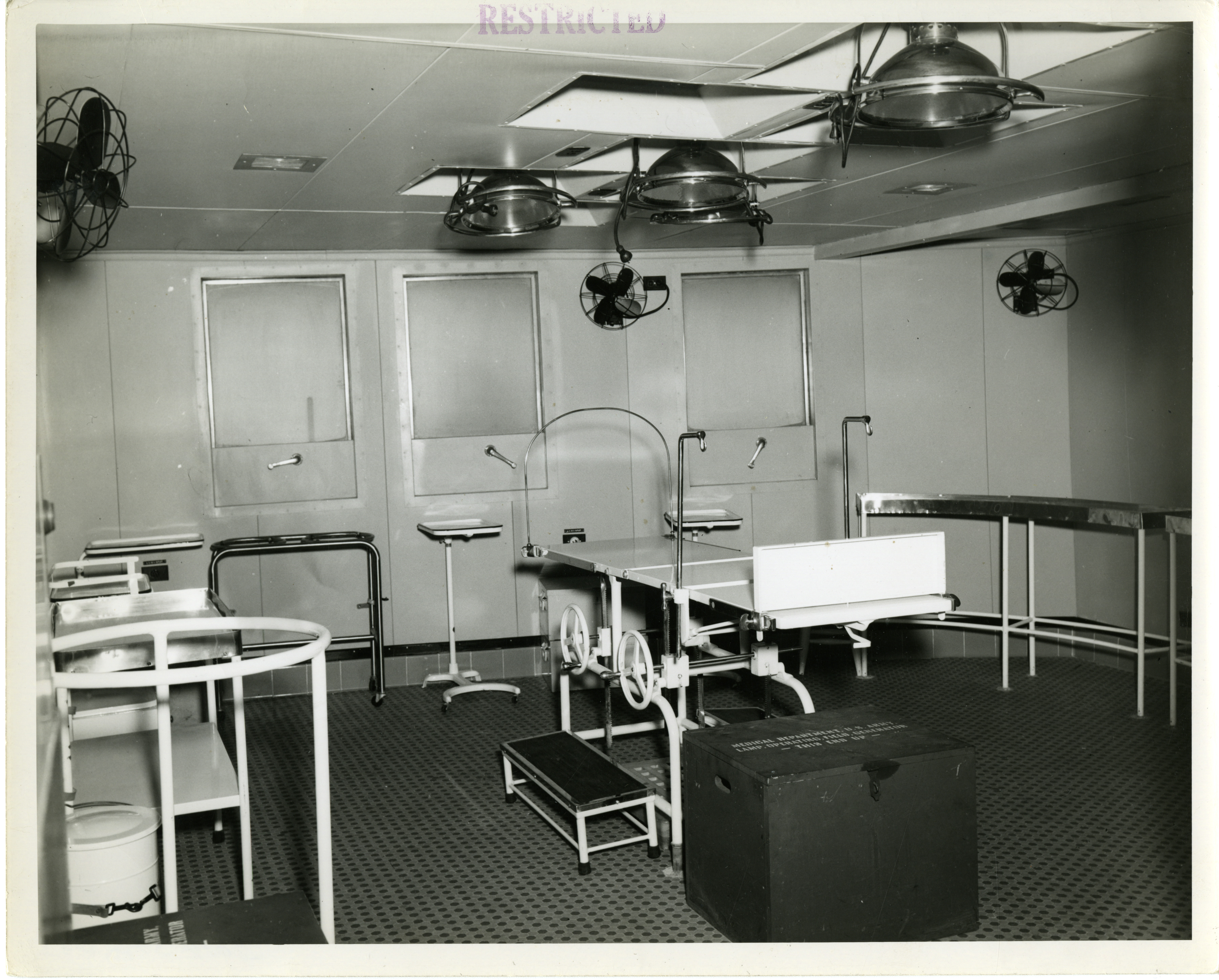This black-and-white photograph, predominantly square with a yellowed white border, depicts a vintage medical operating room, likely from the 1940s or 1950s. The image is marked at the top with a purple or red "Restricted" stamp, indicating its confidential nature. Central to the scene is an old-fashioned operating table, equipped with two wheel cranks for height adjustment and a small step for elevation. Surrounding the table are stainless steel rolling carts, presumably for surgical instruments, and an array of medical equipment. The room's perimeter features several essential fixtures, including three large, round ceiling-mounted spotlights designed for intense illumination during procedures, and three wall-mounted fans to ensure air circulation. The room also includes a green footlocker with a lock, presumably for storing sensitive items. Three shuttered windows at one end of the room, a stainless steel sink to the left, and the black-and-white tile flooring further accentuate the antiquated medical environment of this photograph.